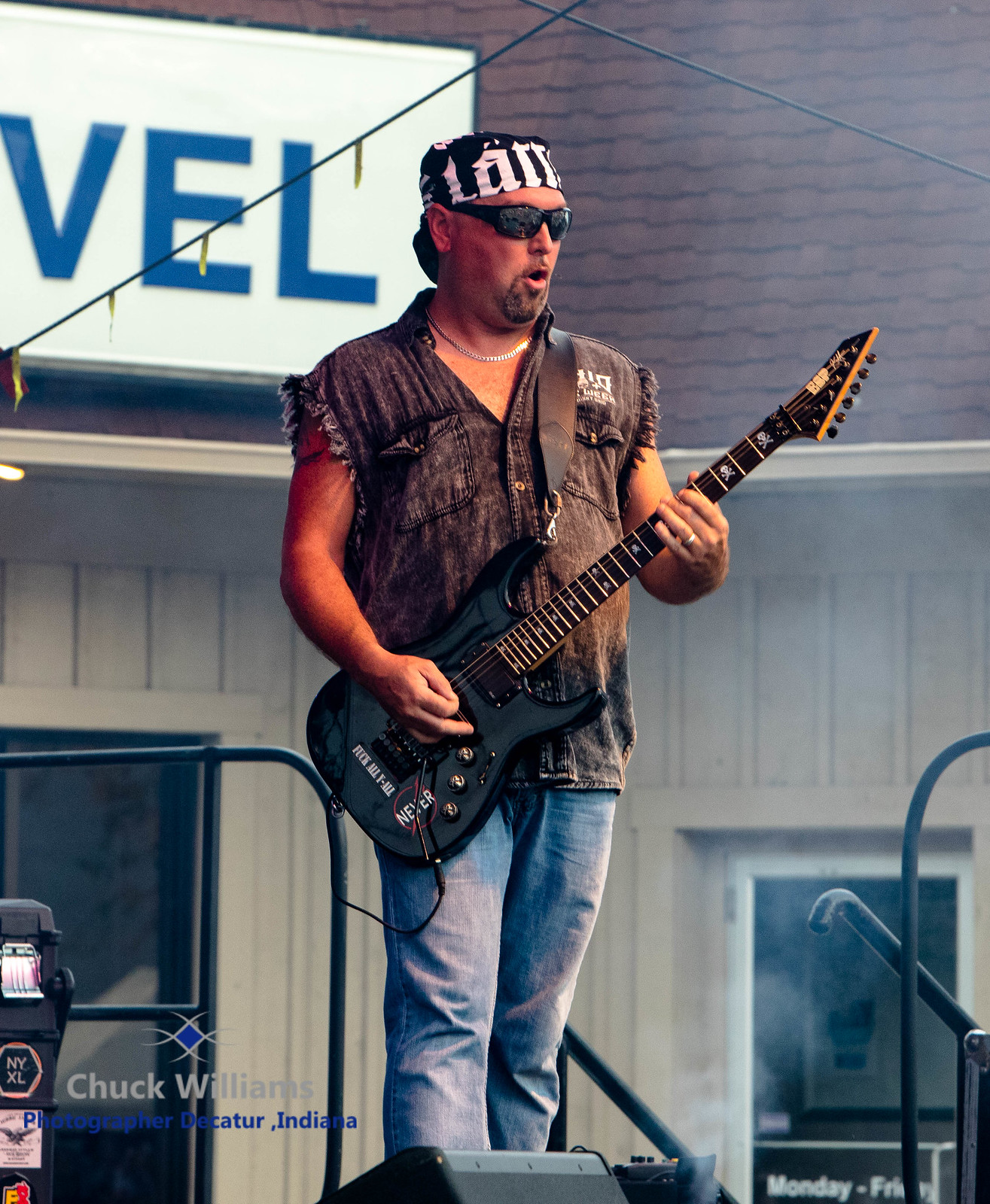The image captures a male guitarist intensely performing on stage during what appears to be a daytime concert. He is dressed in a distinctive outfit: light blue jeans paired with a black, sleeveless denim jacket that is cut off at the arms. He wears dark, black-tinted sunglasses and a black headband adorned with white letters that seem to spell out "L-A-N." A silver chain hangs around his neck, and he sports a small beard. The musician is strumming a black electric guitar and appears to be fully engrossed in his performance. 

The backdrop includes a building with brown shingles and greyish-brown painted walls, featuring a commercial sign with the letters "V-E-L" in blue against a white background. There are windows to both sides of the performer, and the stage is accessible via stairs with black handrails. A hint of smoke seems to rise from the stage area, adding to the concert atmosphere. The bottom left of the image credits "Chuck Williams, photographer, Decatur, Indiana," suggesting it was taken by a professional photographer at an event or concert.